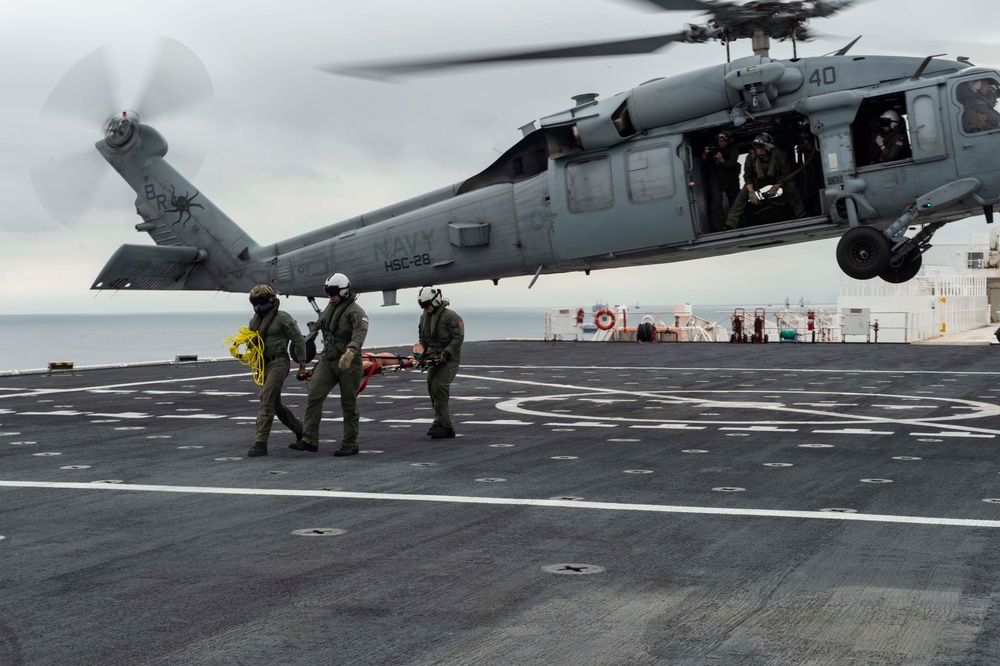This photograph captures a busy moment on the deck of an aircraft carrier at sea. A large, grey, military-style Navy helicopter marked with "Navy HSC-28" is either landing or taking off, its spinning blades creating a blur against the hazy sky. The scene is set against a backdrop of endless ocean, meeting the horizon with a hint of hazy clouds. The deck, an industrial expanse of metal and railings, features a visible helipad where the helicopter hovers just a few feet above the surface. 

In the forefront, three men in helmets and safety gear are walking away from the helicopter. Two of them are carrying an injured person on a backboard, while the third man holds a bright yellow rope. The individuals inside the helicopter look on, possibly after having delivered the injured person. The background reveals additional parts of the ship, a life preserver, and a walkway leading to the main areas of the vessel. This moment, fraught with urgency and precision, underscores the coordinated efforts of a naval emergency operation.